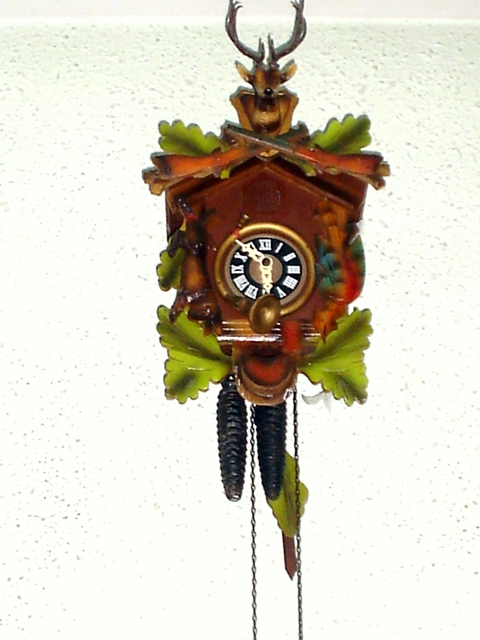This photograph captures a vintage cuckoo clock hanging on a stucco-textured wall that is painted white and partially lime green with dots. The cuckoo clock is designed to resemble a wooden birdhouse and is crafted from dark-tinted wood. The top of the clock features a mounted deer head with prominent antlers, framed by two inverted wooden hunting rifles. The edges and base are adorned with carved green leaves. In the center of the structure is the clock face, which has a black background with white Roman numerals and pearl-white, intricately designed hands. The face is encircled by a gold border and has a distinctive gold circle in the middle. Below the clock face, hanging from brass chains, are two elongated, black pinecone-shaped weights, which are integral to the clock’s mechanism.